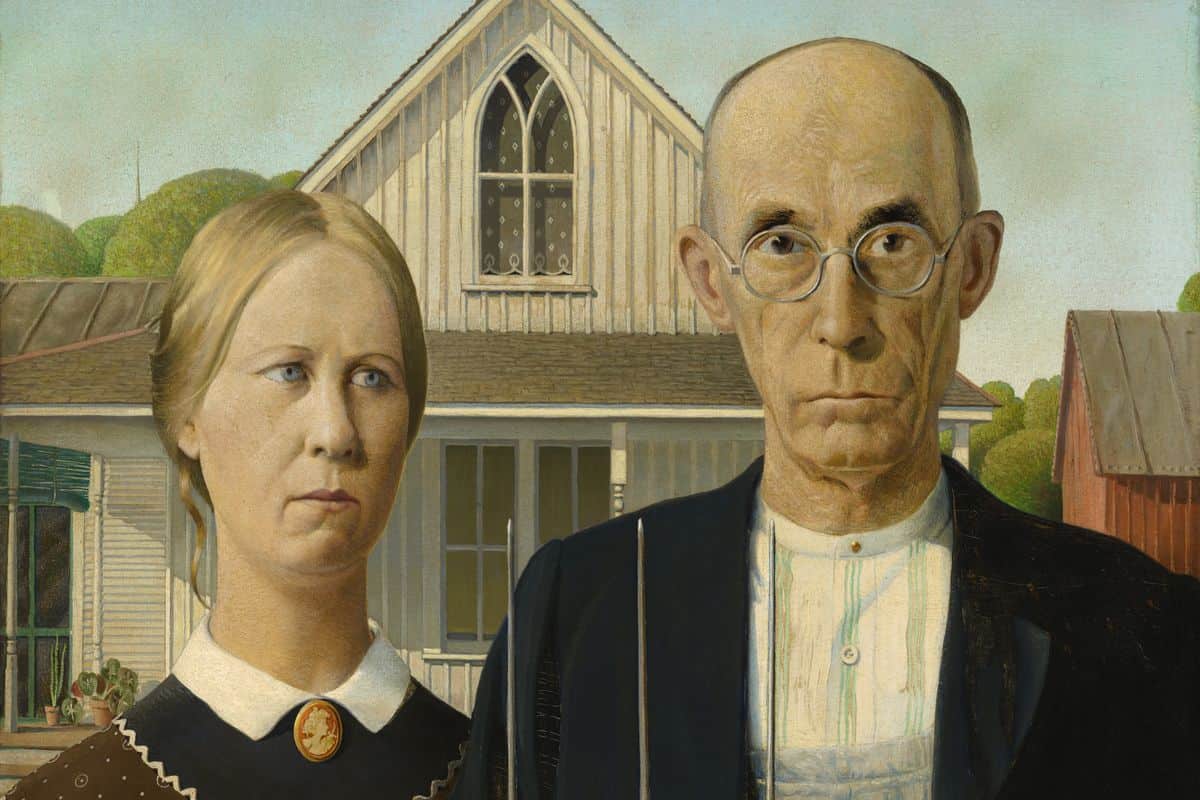This is an image of the famous painting "American Gothic," depicting a stern-looking farmer and a woman, often mistakenly thought to be his wife but actually his daughter. The older man on the right has a thinner build, distinguished by his bald head, silver-rimmed glasses, black eyebrows, and faint wrinkles. He is dressed in a white shirt with vertical green and blue stripes, paired with a dark blue-to-black suit top, and he holds a three-pronged pitchfork. The younger woman to his left has a concerned expression, with bright blue eyes and blonde hair pulled back into a ponytail. She has a long neck, an elongated face, and is wearing a white collared shirt adorned with an Elizabethan-style pendant. Behind them stands a white farmhouse with a distinctive steepled roof and a church-like window, surrounded by a blue sky with soft clouds. Additionally, there's a little red barn with a dark copper-colored steel roof and large green trees adding to the tranquil background.